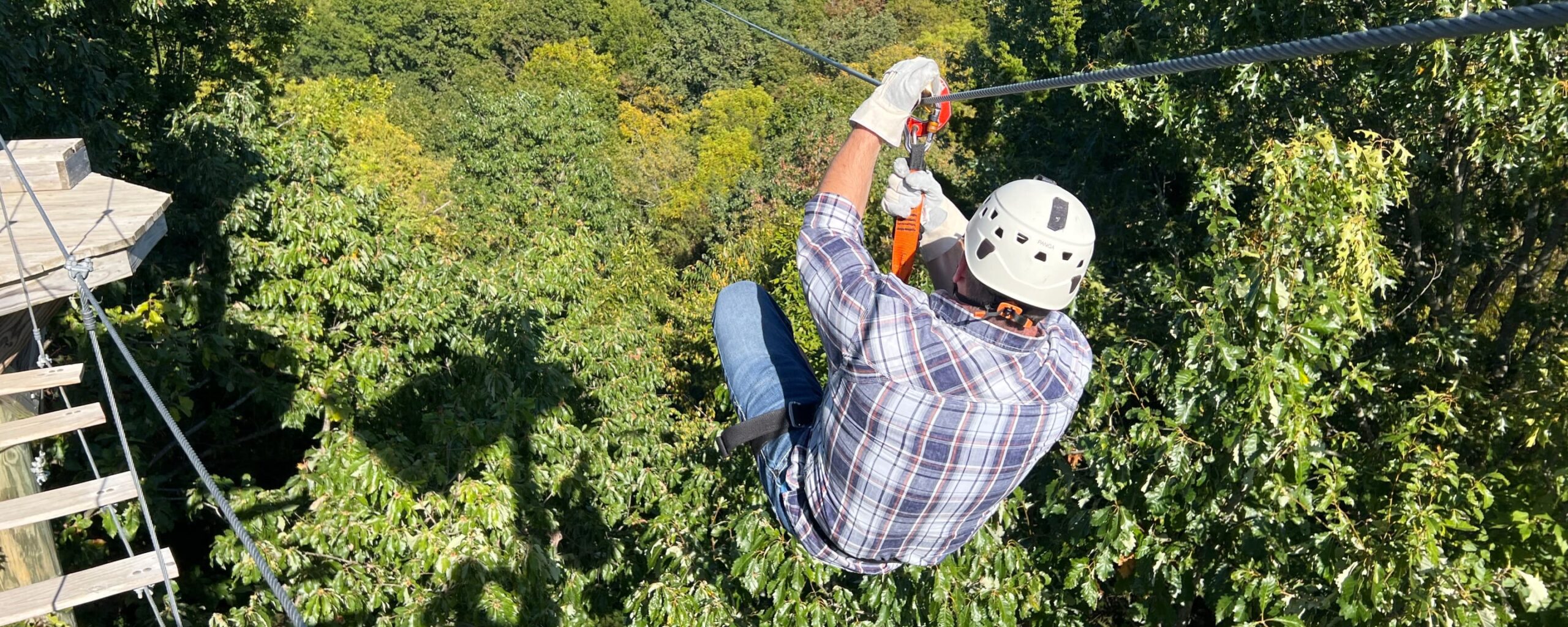The photo captures a man ziplining high above a dense forest, soaring along a solid, professional-grade rope. He is equipped with safety gear, including a white hard hat, gray gloves, and buckles that secure him to the zipline. His striped-collar shirt flutters as he moves swiftly through the air. The zipline is suspended at a great height, elevating him far above a sea of lush treetops, creating a thrilling yet safe adventure. Below, the forest stretches out with a mix of towering trees, making the descent appear perilous if not for his secure harness. A landing station is visible in the distance, marking his destination as he zips through this verdant canopy, clearly enjoying the exhilarating ride.